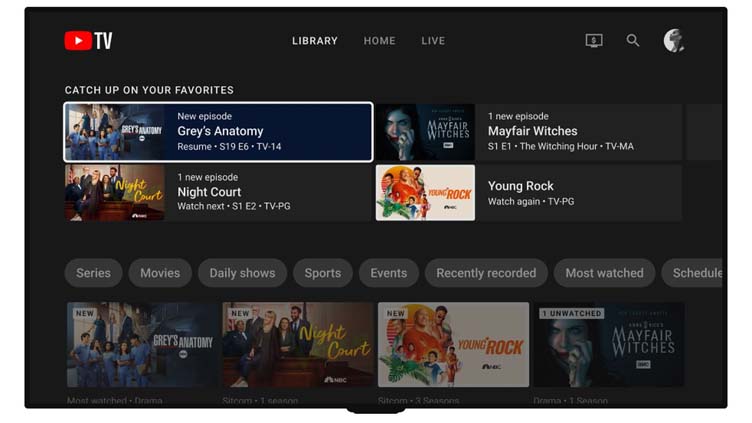This image is a detailed screenshot of the YouTube TV interface, characterized by a dark gray background. In the top left corner, the prominent YouTube logo is followed by the white letters "TV." Central navigation options include "Library," "Home," and "Live," with "Library" bolded to indicate the current selection. The top right corner features a computer icon with a dollar sign inside a magnifying glass, alongside a circular grayscale thumbnail of a Black woman against a white background.

Beneath this, on the left-hand side, a title reads "Catch up on your favorites," followed by a list of TV shows with viewing options:

- "Grey's Anatomy": new episode, "Resume S19E6," rated TV-14.
- "Mayfair Witches": new episode, "S1E1, The Witching Hour," rated TV-MA.
- "Night Court": new episode, "Watch Next S1E2," rated TV-PG.
- "Young Rock": "Watch Again," rated TV-PG.

Below these, a set of grey buttons with white text offers additional viewing categories such as "Series," "Movies," "Daily Shows," "Sports," "Events," "Recently Recorded," "Most Watched," and "Scheduled."

At the bottom of the screen, thumbnails of shows like "Grey's Anatomy," "Night Court," "Young Rock," and "Mayfair Witches" are displayed once more for easy access.